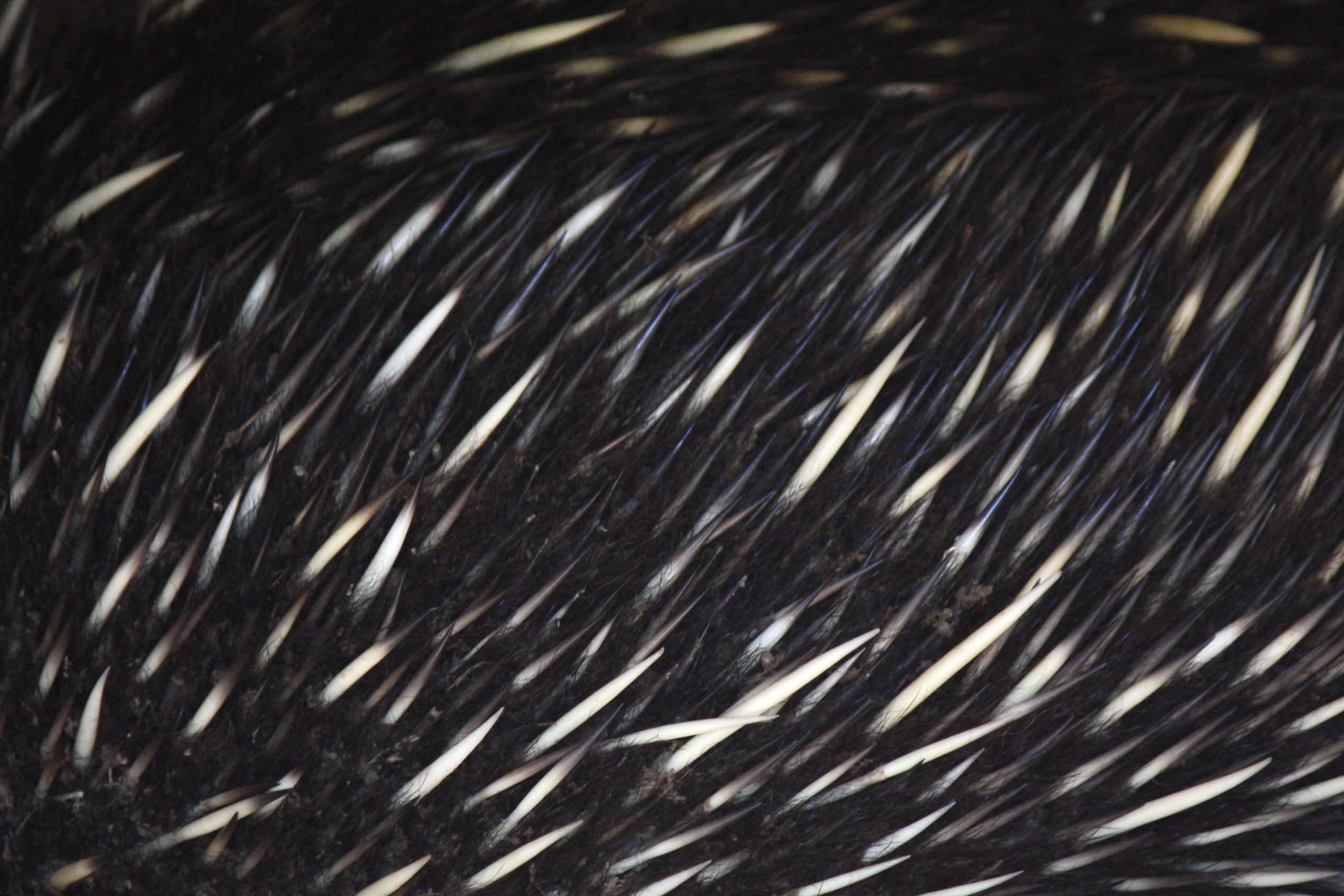The color photograph presents an extreme close-up of black strands meticulously laid out, with light subtly glinting off certain areas. These strands could be quills, resembling porcupine quills with black bases and white tips, as they are notably sharp and well-arranged in a diagonal pattern from the bottom left to the top right. Alternatively, the strands may evoke the appearance of reeds or aquatic creatures viewed from above, as there is a gradient in thickness from one end to the other, akin to how reeds might bend in the wind or fish might swim in a coordinated direction. The strands are set against a predominantly black background with occasional glimmers of light adding depth and intricacy, making it both detailed and enigmatic.